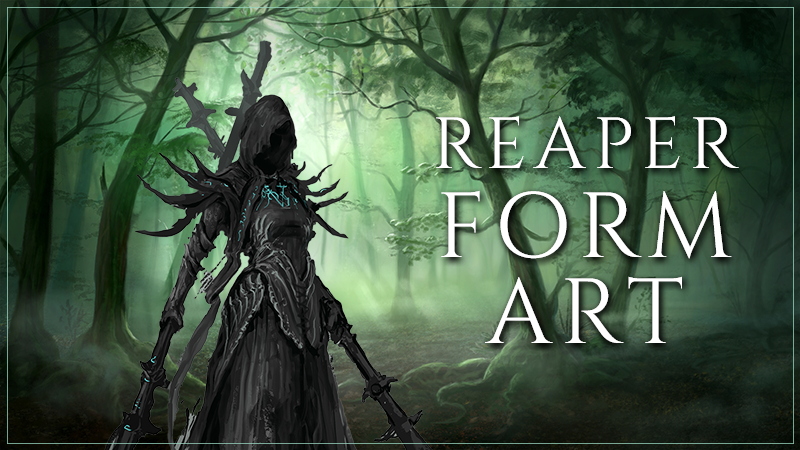This image, seemingly video game or AI-generated art, depicts a mysterious, wood-dwelling Reaper-like entity. The rectangular artwork, oriented horizontally, showcases a dark, ominous figure set against a forest backdrop. The creature, possibly a wood elf or woodland spirit, is cloaked in a long, dark robe with a hood that conceals its face, exuding a faceless, sinister aura. Strapped to its back are two sword-like weapons, and its chest features light blue lines, indicative of some form of armor. The shoulders are accentuated with skeletal, demon-like wings or spikes.

The forest setting is both eerie and beautiful, bathed in a soft, green light that filters through the leafy canopy. The trees, with dark green trunks and leaves, seem to lean towards the light source, adding to the mystical atmosphere. The entire scene is cast in shades of black, gray, and green, with the light creating a hazy glow, particularly towards the middle and left of the image. In white font on the right-hand side, the words "Reaper Form Art" are prominently displayed, further emphasizing the character's grim and otherworldly nature. The image manages to blend elements of fantasy and darkness, making it reminiscent of a Dungeon and Dragons-inspired fantasy world.